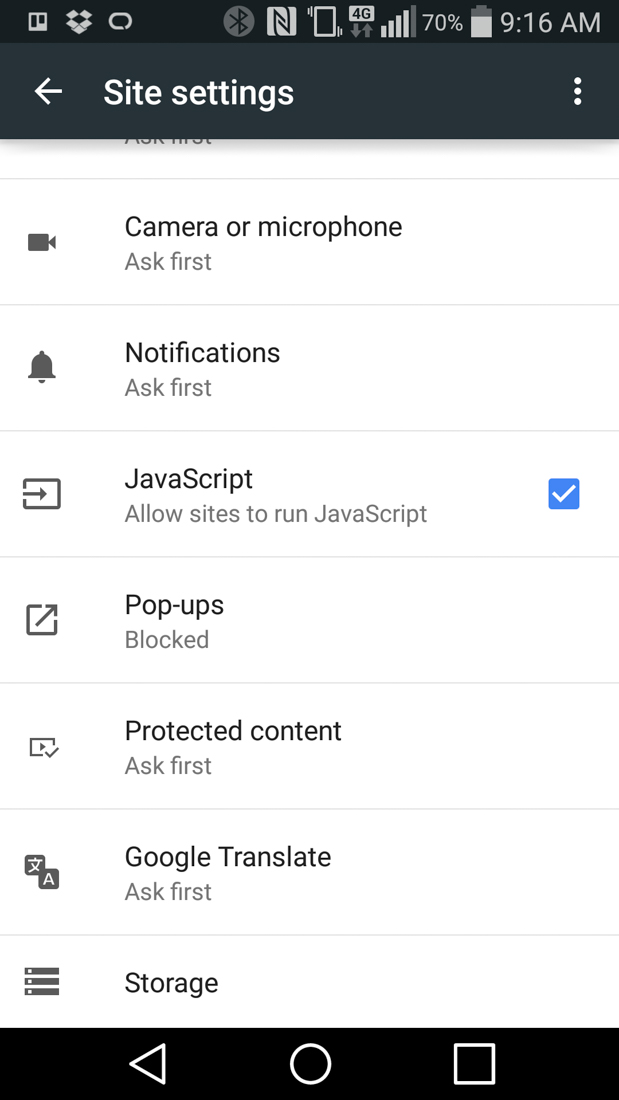This image is a screenshot from a mobile device displaying the "Site Settings" screen. At the top of the screen, the title "Site Settings" is prominently featured. The status bar is visible at the very top-left corner, showing several icons: notifications, Bluetooth, 4G connection, battery at 70%, and the time, 9:16 a.m.

The settings listed on the screen under "Site Settings" include:

1. **Camera** - "Ask first"
2. **Microphone** - "Ask first"
3. **Notifications** - "Ask first"
4. **JavaScript** - "Allow sites to run JavaScript" (this setting has a blue checkbox next to it)
5. **Pop-ups** - "Blocked"
6. **Protected content** - "Ask first"
7. **Google Translate** - "Ask first"
8. **Storage** - Simply labeled as "Storage" with no additional setting provided.

This screenshot appears to be taken from an older Android device, inferred from the layout and design of the buttons at the bottom of the screen.